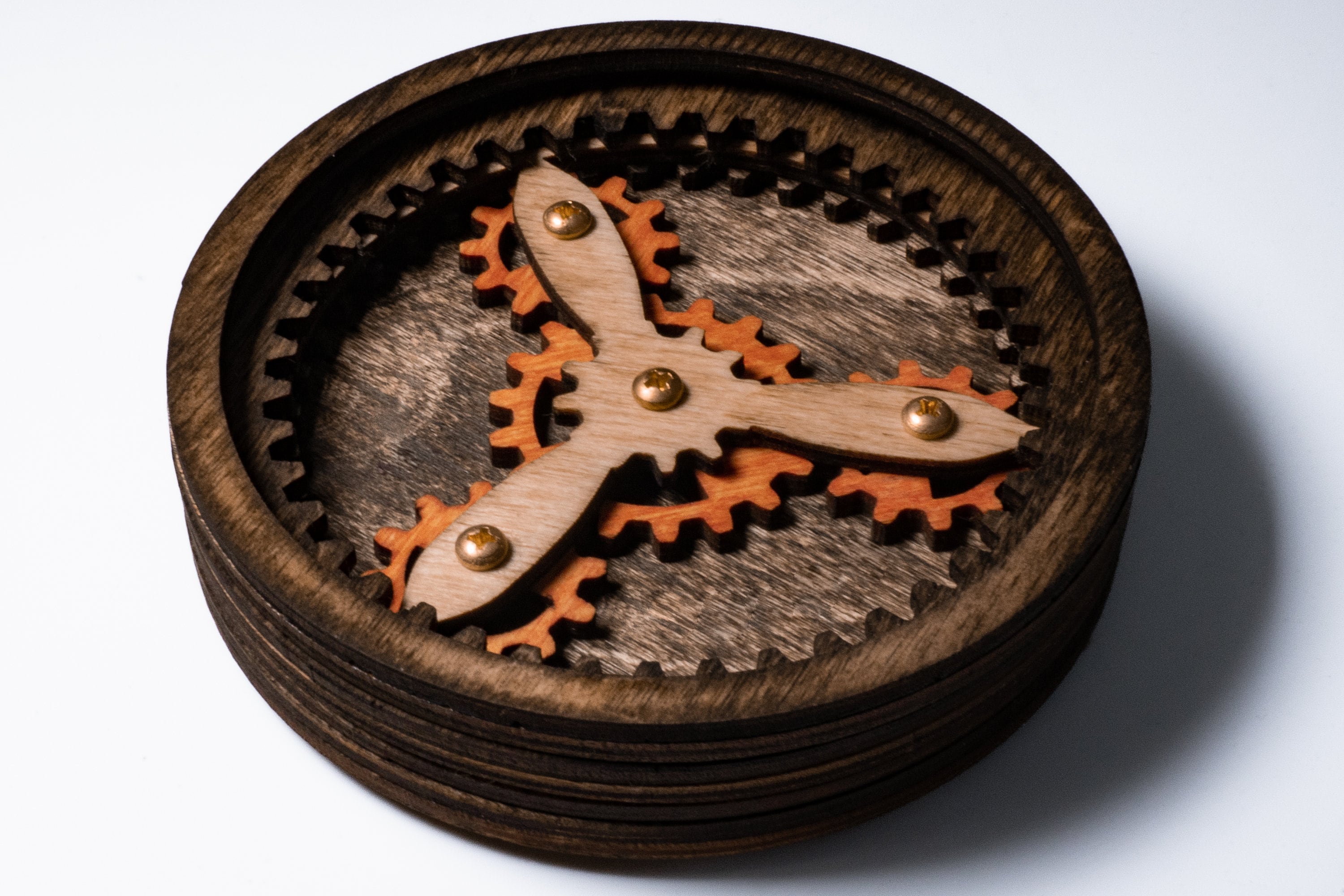This detailed photograph features a meticulously carved, dark chocolate brown wooden coaster-like object with a round shape and an indent extending a few inches deep into its center. The inner sides of this indentation are intricately lined with jagged, gear-like ridges. Nestled within the recessed area are four orange wooden gears: one larger central gear surrounded by three smaller gears positioned equidistantly around it, forming a triangular pattern. A wooden propeller-like piece, secured by screws at three points and in the middle, rests atop these gears, enabling them to interact and rotate. While its precise function remains unclear, it appears to be a decorative piece, perhaps intended as an intriguing and artistic coaster for a drink.